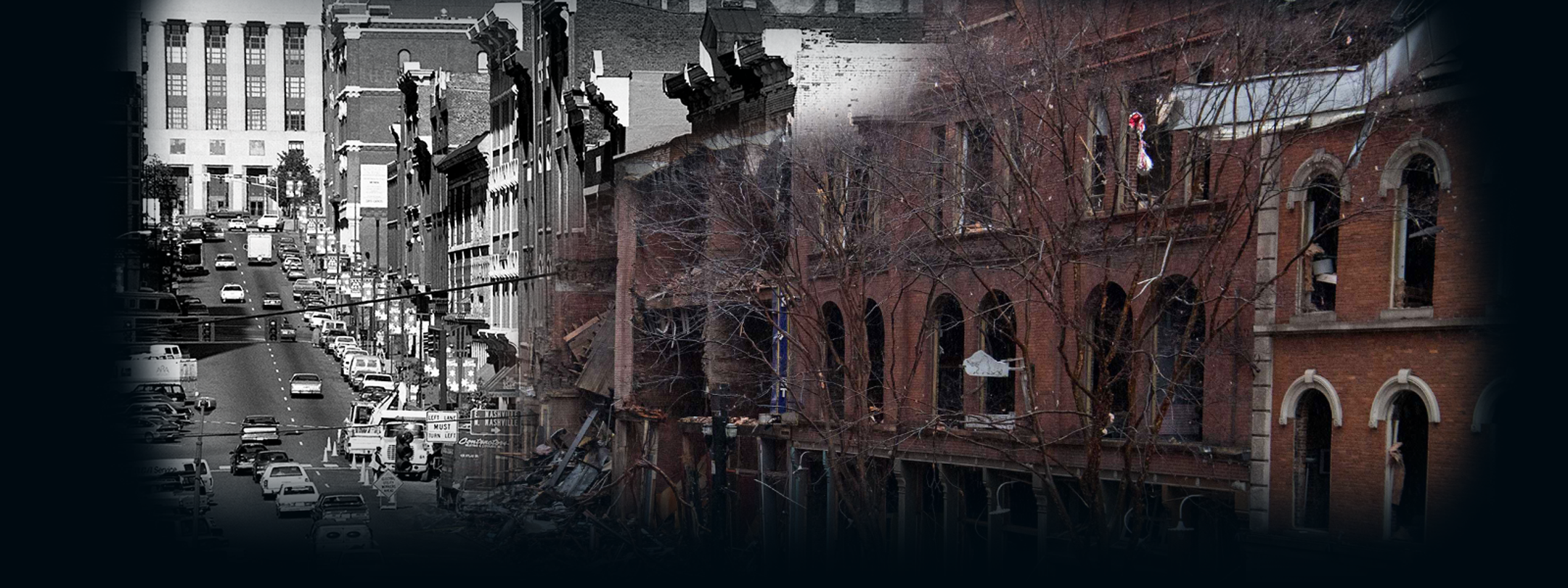This photograph showcases a city street scene, featuring a striking combination of two time periods. The right side of the image is in vivid color, depicting a large red brick building that appears to be intact and modern. In contrast, the left side of the photograph is in black and white, revealing the same street and building but from an earlier era. This portion shows some wear, with parts appearing abandoned, demolished, or under construction, evident from the visible window cutouts lacking glass and sections seemingly crumbling into the street. The cars on the road bridge the two eras, showcasing a seamless blend between the historical and contemporary views. The borders of the photograph are marked with a black vignette, enhancing this juxtaposition of time. The image is devoid of text and people, but leafless trees and modern cars are present, hinting at a cold season and making the contrast between the two halves even more poignant.